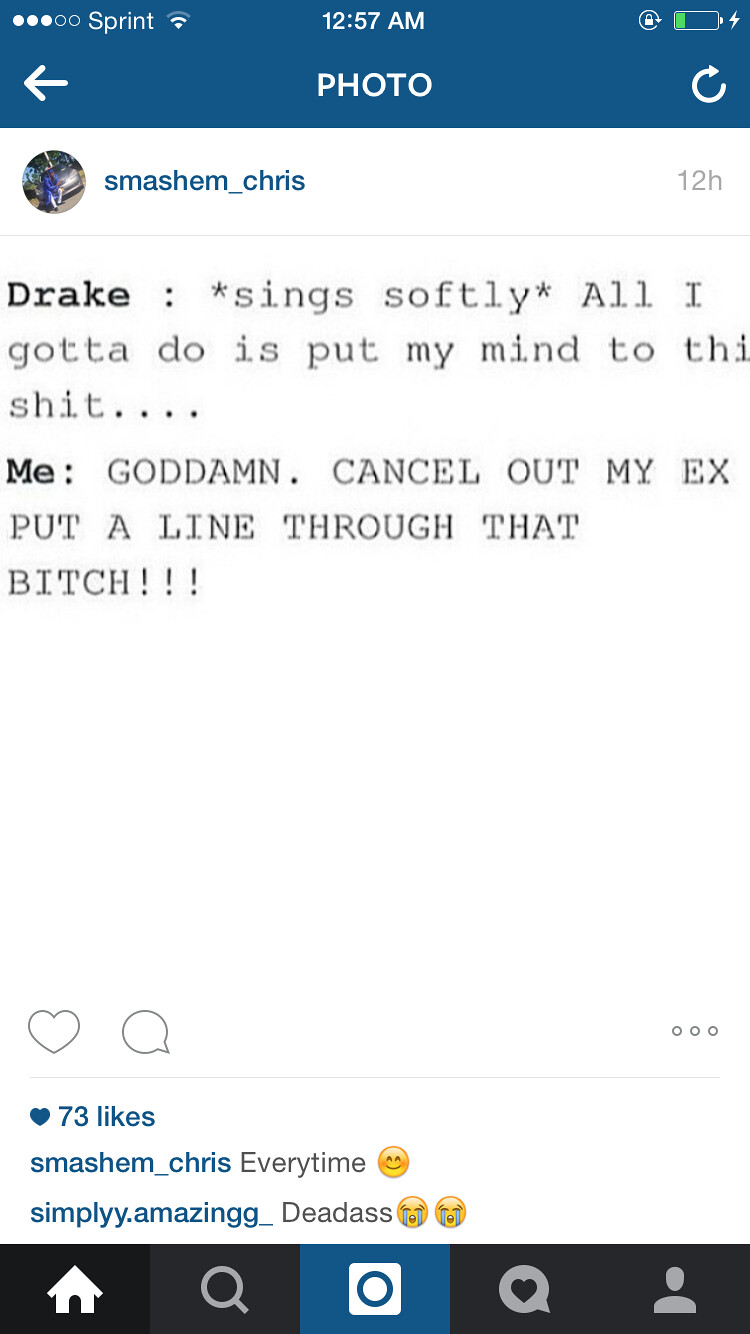This is a detailed screenshot taken from an iPhone displaying a social media post. The top of the screen shows the status bar with "Sprint", the time "12:57 AM", and battery indicators. Below that, a blue navigation bar contains a back arrow on the left, the word "Photo" in the center, and a refresh icon on the right. The post is from "Smash Him Chris", whose profile picture is in a small circle next to his name. The post reads: "Drake. Sing softly. All I gotta do is put my mind to this shit. Me, goddamn, cancel out my ex, put a line through that bitch." This caption references a popular song with specific lyrics. The post has 73 likes and a comment from "Smash Him Chris", stating "every time" followed by a smiley face emoji. A reply from "simply.amazing" underneath reads "dead ass" accompanied by two crying face emojis. At the bottom, the screen features navigation icons for home, search, camera, likes, and profile, all set against a blue, white, black, green, and gray color scheme. The entire image is a well-lit and clear screenshot highlighting the user interface and interactions on this social media app.